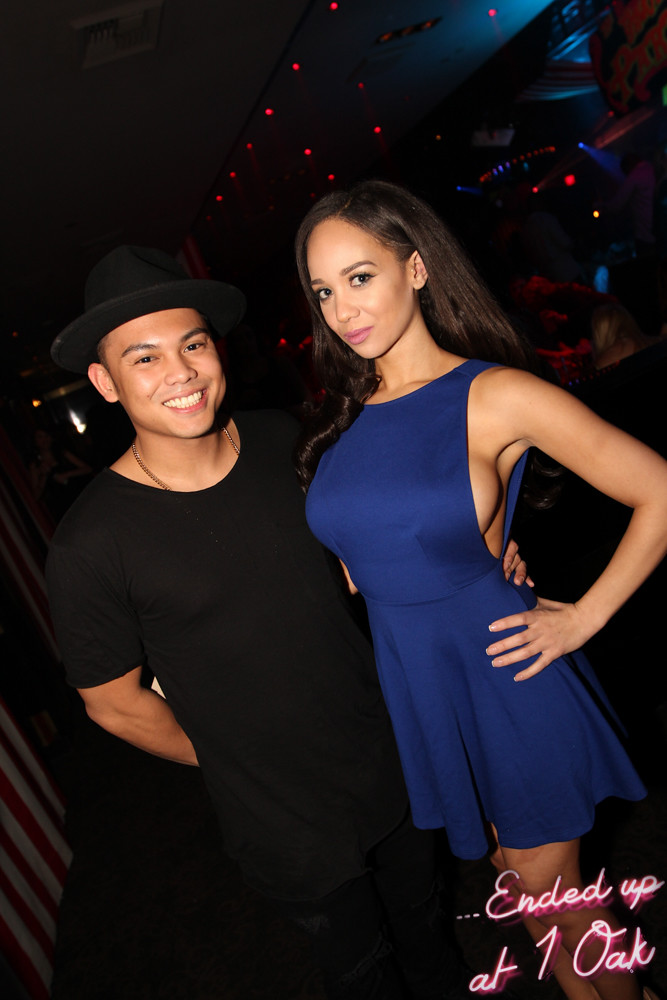This color photograph captures a young man and woman at a nightclub, presumably called One Oak, as indicated by the white and pink script lettering in the bottom right corner. The man, positioned on the left, is dressed entirely in black, including a T-shirt, pants, and a hat, and accessorized with a gold necklace. He smiles warmly while his left arm wraps around the waist of the woman standing to his right. The woman, wearing a short blue dress, has long dark brown hair and strikes a confident pose with her left hand on her hip. She also sports a slight smile as they both look directly into the camera. The background of the photograph is predominantly dark, with a few small red, blue, and yellow lights suggesting the lively atmosphere of a nightclub.